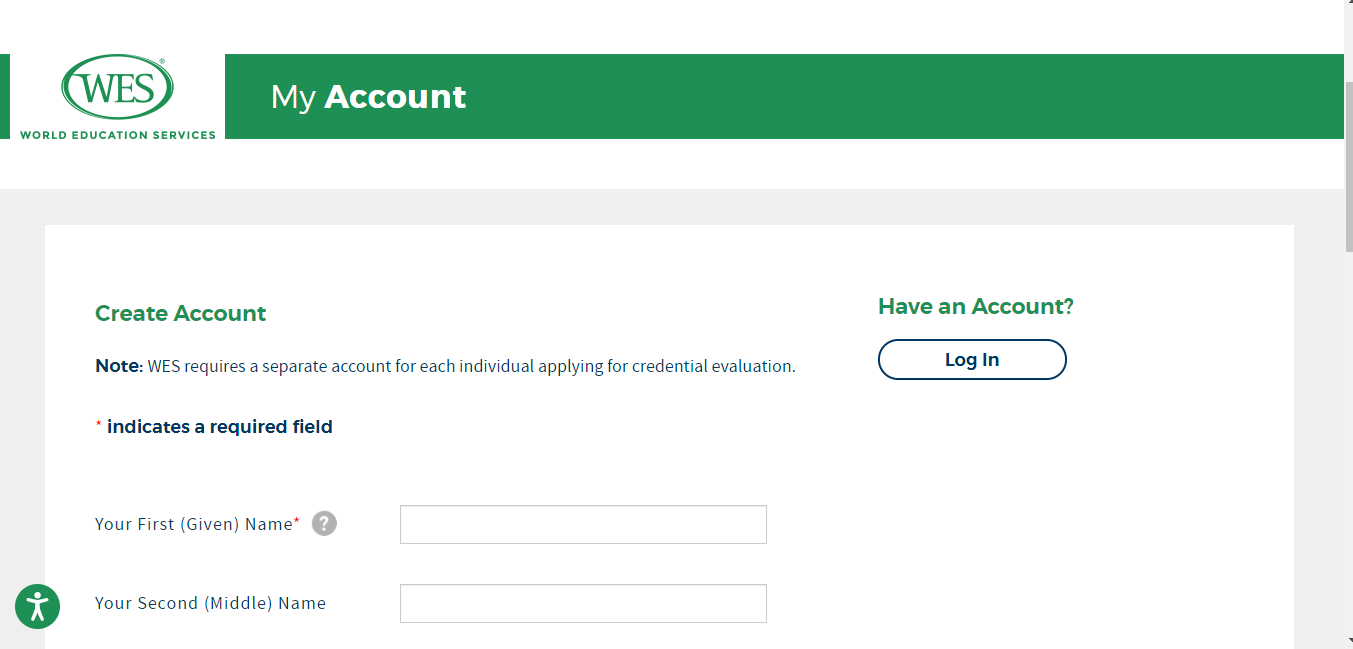This screencap showcases the login page of the World Education Services (WES) website. Prominently positioned in the top-left corner is the WES logo, consisting of the capital letters "W-E-S" encased within a green circle, accompanied by the organization's name written in green text beneath the logo. The page is headed by a green navigation bar labeled "My Account."

Below the navigation bar, the website features a white background typical of most web pages. Users have the option to create a new account or log in if they already have one, with the login button conveniently located on the right-hand side. For new users, there are fields to input personal information such as names. A notable detail is a message stating that WES requires a separate account for each individual applying for a credential evaluation.

In the lower left-hand corner of the page, a green circle containing a person icon highlights an accessibility feature, ensuring the website is user-friendly for individuals with disabilities.